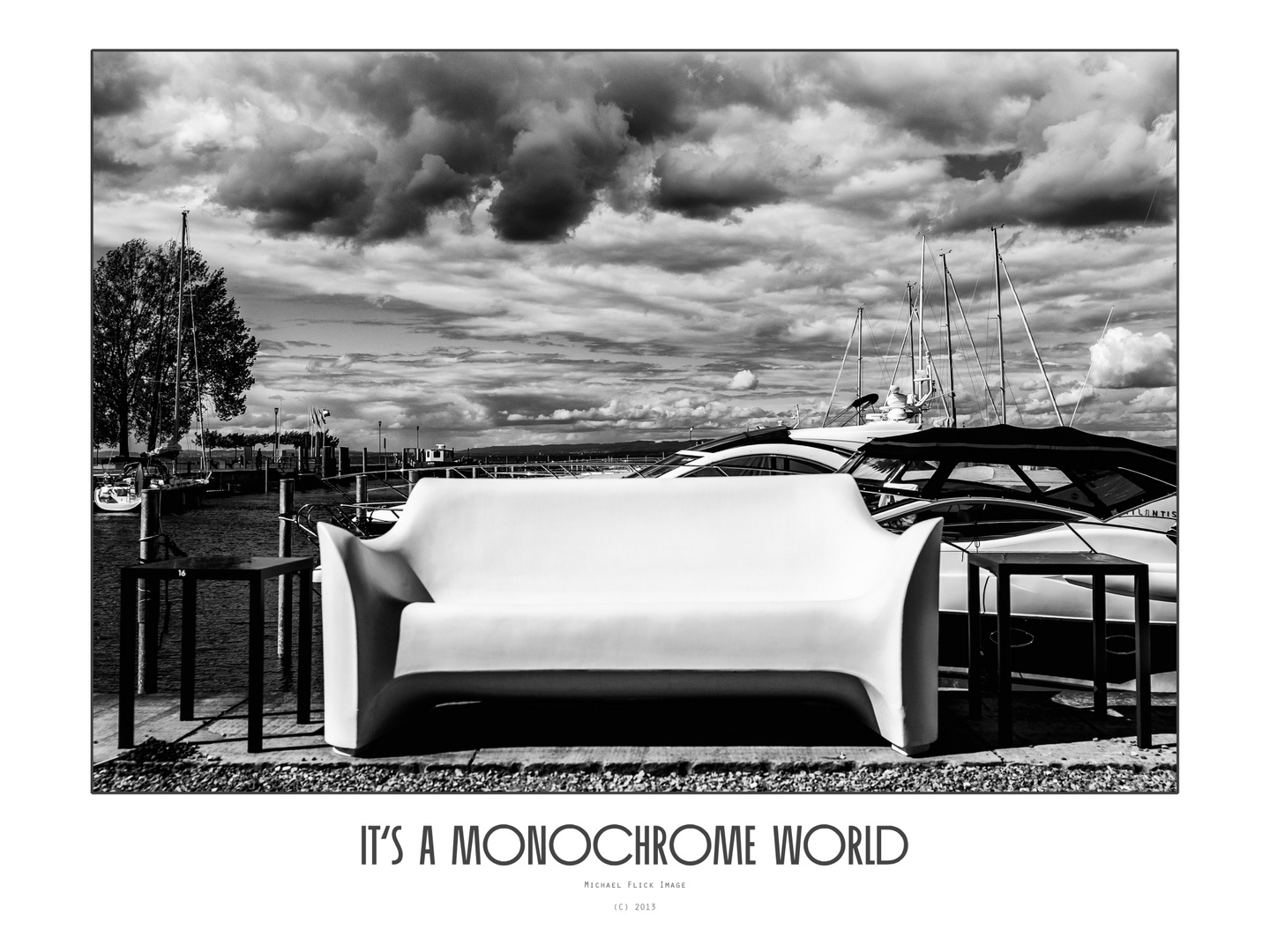In this high-definition black and white image, a uniquely carved bench designed to resemble a couch is the central focus. This outdoor piece of furniture, seemingly made from a single solid material, features sharp-looking curved armrests and is situated on a stone tile platform. Positioned overlooking a marina, the bench is flanked by two glossy black side tables, contributing to the minimalist aesthetic. The marina, filled with multiple yachts and sailboats, stretches out behind the bench, with trees visible in the distance. The sky above dominates the top half of the image, filled with dramatic, dark clouds on an overcast day. At the bottom of the image, black text reads, "It's a monochrome world," emphasizing the complete spectrum of black, white, and gray shades. This striking photograph, taken in 2013 by Michael Flick, evokes a sense of serene contemplation in its carefully balanced composition and stark monochromatic palette.